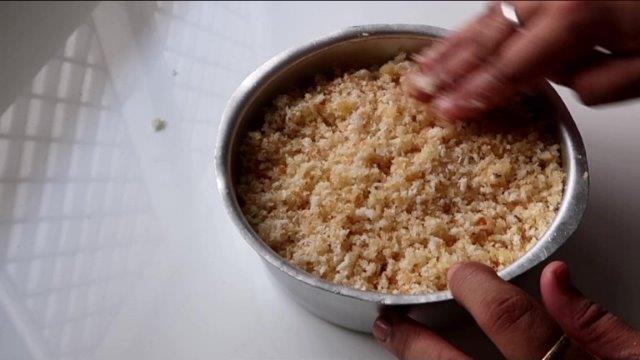The image features a silver bowl placed on a pristine white surface. The bowl's interior is filled with a brownish-white mixture, which could be rice, rice krispies, crumbled bread, or a seasoned blend. The weight and texture of the mixture are evident as part of it sticks to the fingers maneuvering inside the bowl.

A person's right hand emerges from the bottom right corner of the image, extending their thumb, index finger, and the tip of their ring finger towards the bowl. The index finger, adorned with a silver ring, hovers over the bowl, perhaps engaged in a tactile assessment of its contents. Meanwhile, the left hand descends from the top right of the frame, with three fingers tightly grouped together, delving into the bowl's mixture. The substance clings to these fingers as if they have been used to stir or mix the contents vigorously. This hand also sports a silver ring on the middle finger, while the thumb remains curled beneath the hand.

The white surface beneath the bowl reflects light, creating an intricate pattern of crisscrossing vertical lines. The person's dark skin contrasts sharply against the light background and the metallic sheen of the bowl, highlighting their engagement with the bowl's contents.